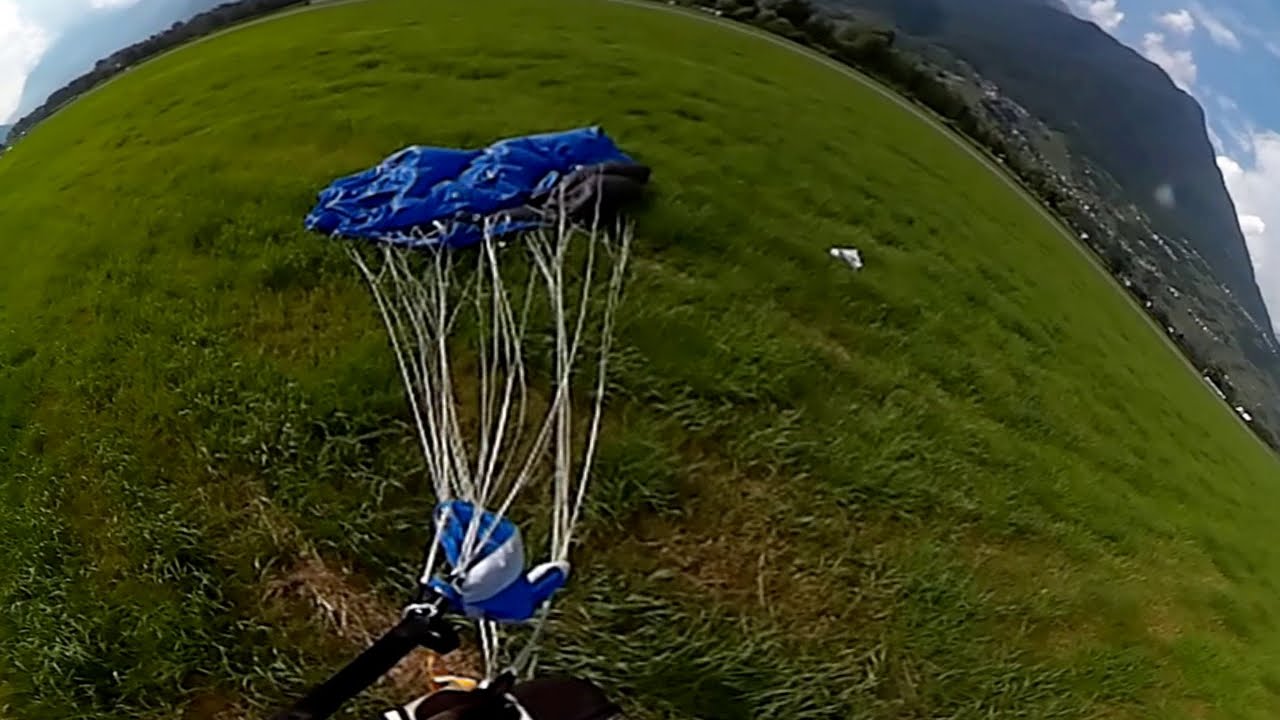The image depicts a vividly green grassy area in the foreground with a collapsed navy blue parachute spread out on the ground. The parachute features white strings and darker blue closures. The grass appears oddly curved, which adds to the overall distortion of the image, making the landscape look spherical. This distortion is further seen in the background, where the mountains and trees arc around the horizon in an unusual manner. On the left side, parts of the mountains seem obscured by clouds. There is a narrow path or roadway visible on the horizon, behind which stands a row of trees. Beyond the trees are some buildings, followed by the arcing mountains and a clear blue sky with scattered white clouds, primarily clustered in the right-hand corner. The scene gives the impression that it might have been captured from a body cam during a parachuting activity, with the parachute's landing recorded at the moment of the still shot.